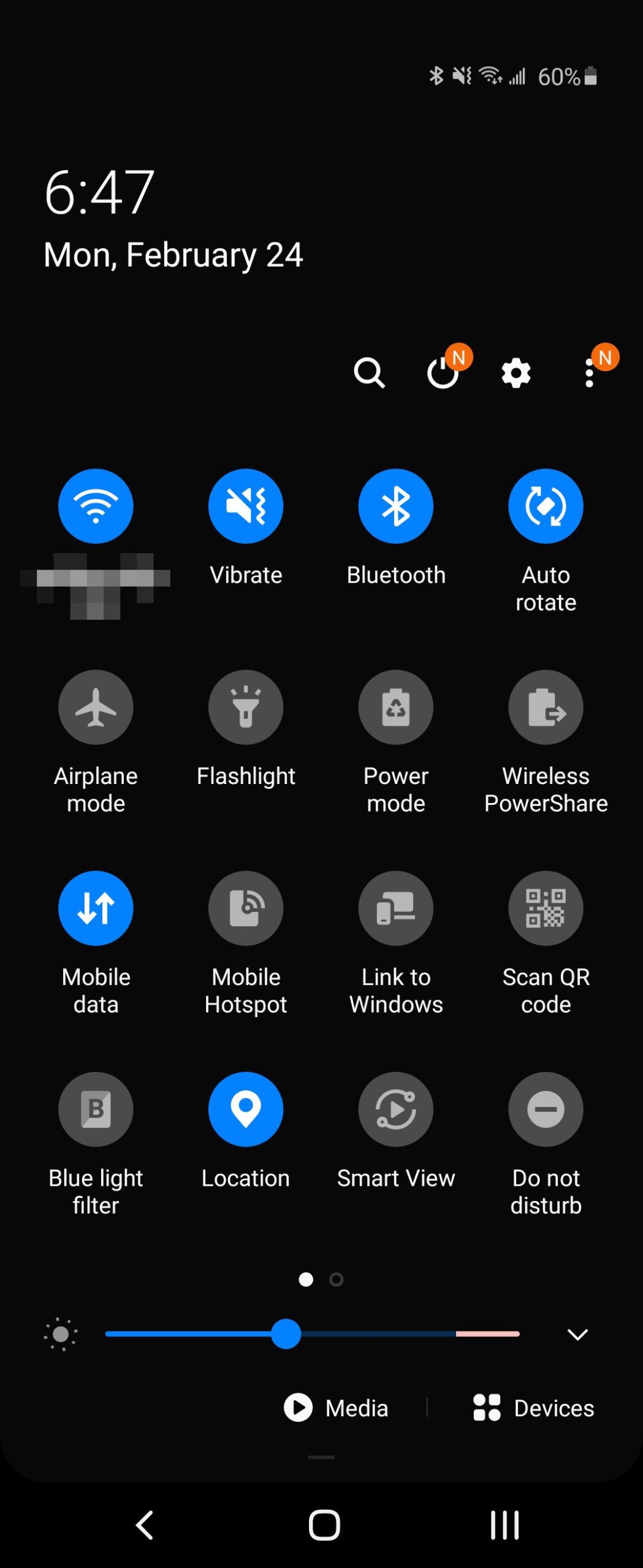Title: Detailed Interface Screenshot on February 24th

The image captures a detailed interface layout, showcasing various system icons and buttons on a digital screen. 

In the top-left corner, the timestamp reads "6:47, Monday, February 24th." Below this, on the right side, a series of functional icons are aligned horizontally: a magnifying glass representing the search function, a power symbol enclosed in an orange circle labeled "N," a cogwheel for settings, and three vertical dots within another orange circle also labeled "N."

Further down, several system status symbols are visible. These include a Wi-Fi icon and adjacent blurred text, a speaker symbol marked "vibrate," a Bluetooth icon with the text “Bluetooth,” and an auto-rotate icon depicting a rotating phone.

Continuing through the interface are icons representing:
- Airplane Mode (a simple airplane symbol)
- Flashlight (depicted by a flashlight)
- Power Mode (an image of a battery)
- Wireless Power Share (a battery with an arrow pointing right)
- Mobile Data (arrows pointing downward and upward)
- Mobile Hotspot (a phone with the Wi-Fi signal)
- Link to Windows (an icon of a phone and laptop)
- QR Code Scan (an image of a QR code)
- Blue Light Filter (a square labeled "B")
- Location (a location pin icon)
- Smart View (an emblem with a swirling arrow enclicting a circle)
- Do Not Disturb (a circle within another circle with minor text visible)

At the lower section of the screenshot, a brightness adjustment bar is positioned in the middle, and underneath this bar, labels read "Media" and "Devices."

Each icon is neatly displayed, providing quick access to the device’s functionalities. Despite some blurred text, the image effectively conveys a comprehensive view of the device's interface at the specified date and time.